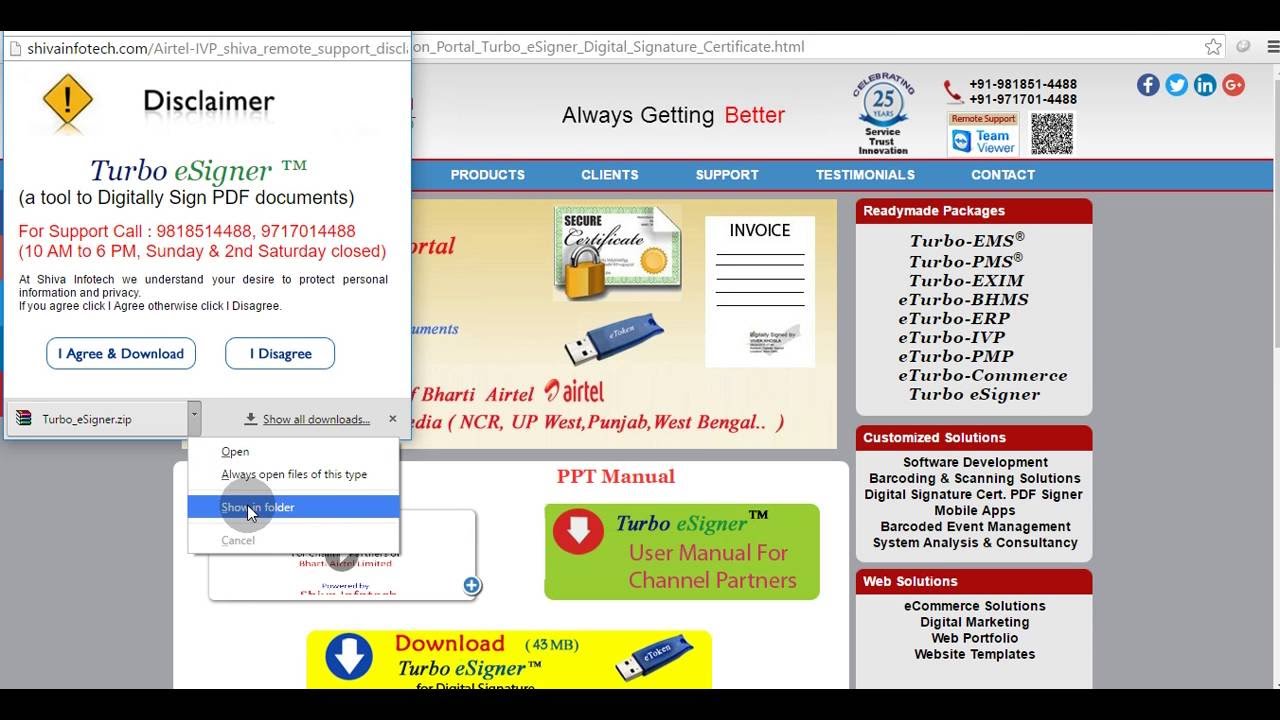In this image, a website interface is displayed prominently. On the left side of the screen, there's a disclaimer box containing text about the Turbo e-Signer™ tool, which is used to digitally sign video documents. The disclaimer provides support contact information with the numbers 981 8514 488 and 97170 14488, and specifies support hours from 10 am to 6 pm, with closures on Sundays and the 2nd Saturday of each month. The text emphasizes the importance of protecting personal information and privacy, instructing users to click "I agree" if they consent, or "I disagree" if they do not. Below the disclaimer, dialog boxes with "I Agree and Download" and "I Disagree" options are visible. Notably, the mouse cursor is positioned over the "Show in folder" option. The image also includes a caption that reads "Always getting better" in smaller text.